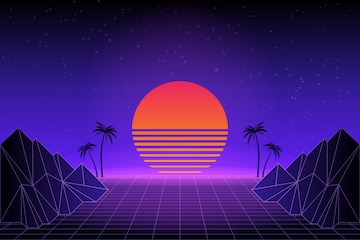This detailed digital render showcases a retro-style, aesthetically pleasing landscape reminiscent of a computer screen background. Dominating the center is a vibrant orange sun, its top half a solid orange gradient into red, while the bottom half is segmented into horizontal orange stripes separated by thin purple lines, creating a unique, split appearance. Surrounding the sun is a striking background of deep black and dark blue sky, dotted with scattered white stars. 

In the foreground, a holographic, gridded floor with neon purple stripes stretches out, lending a dynamic depth to the scene. The horizon features a subtle neon-glowing purple line. Flanking the sun on each side are silhouetted triangular mountains in dark navy blue, outlined in purple, enhancing their digital depth. Adjacent to these mountains, identical black palm trees stand, with a tall palm tree beside a slightly smaller one on each side.

This meticulous blend of vibrant colors and geometric elements creates a visually captivating and immersive retro-futuristic landscape.